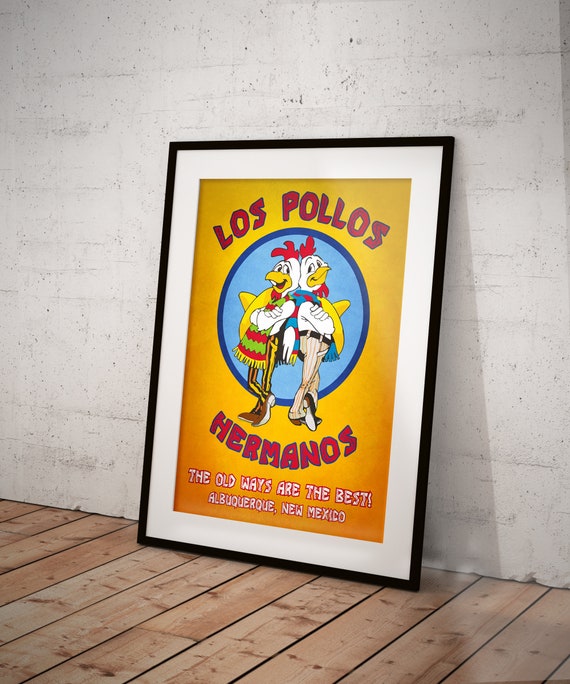The image features two anthropomorphic cartoon chickens standing side by side. Above their heads, a sign reads, "Los Pollos Hermanos - The Old Ways Are The Best," with a subtitle indicating the location: Albuquerque, New Mexico. The chickens have avian heads but human-like bodies. The chicken on the left sports a colorful green, red, and yellow scarf, paired with yellow and black striped pants and brown shoes. Meanwhile, the chicken on the right is dressed in a white shirt and beige striped pants. Both characters are depicted with cheerful expressions, emphasizing a light-hearted and playful atmosphere.